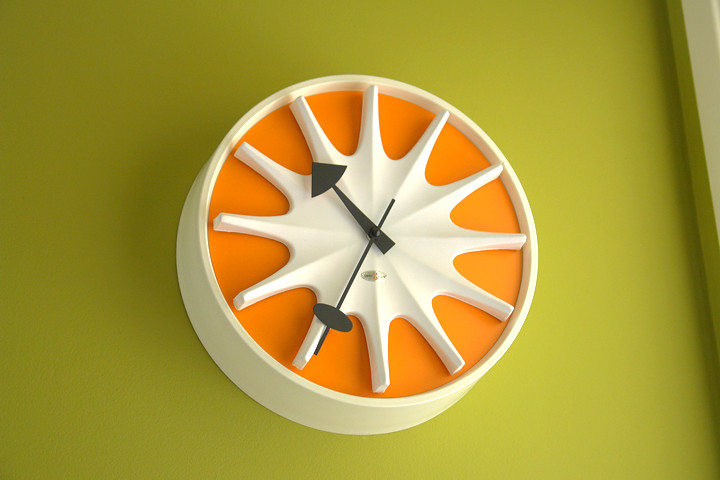This photograph features an excellently captured image of a lime green wall, which serves as a vibrant backdrop. Prominently displayed at the center of the wall is a white circular clock. The clock's face is striking in its bold orange color and is overlaid with a large, geometric white pattern that adds an artistic touch. The clock lacks traditional Roman numerals or numbers, opting instead for distinctive, spiky white hour markers. In the center of the geometric design, two black hands indicate the time with precision. Just below these hands, a silver sticker is visible, adding a subtle yet intriguing detail. Light and shadow interplay at the top of the clock, further enhancing the dimension and visual appeal of this high-quality image.